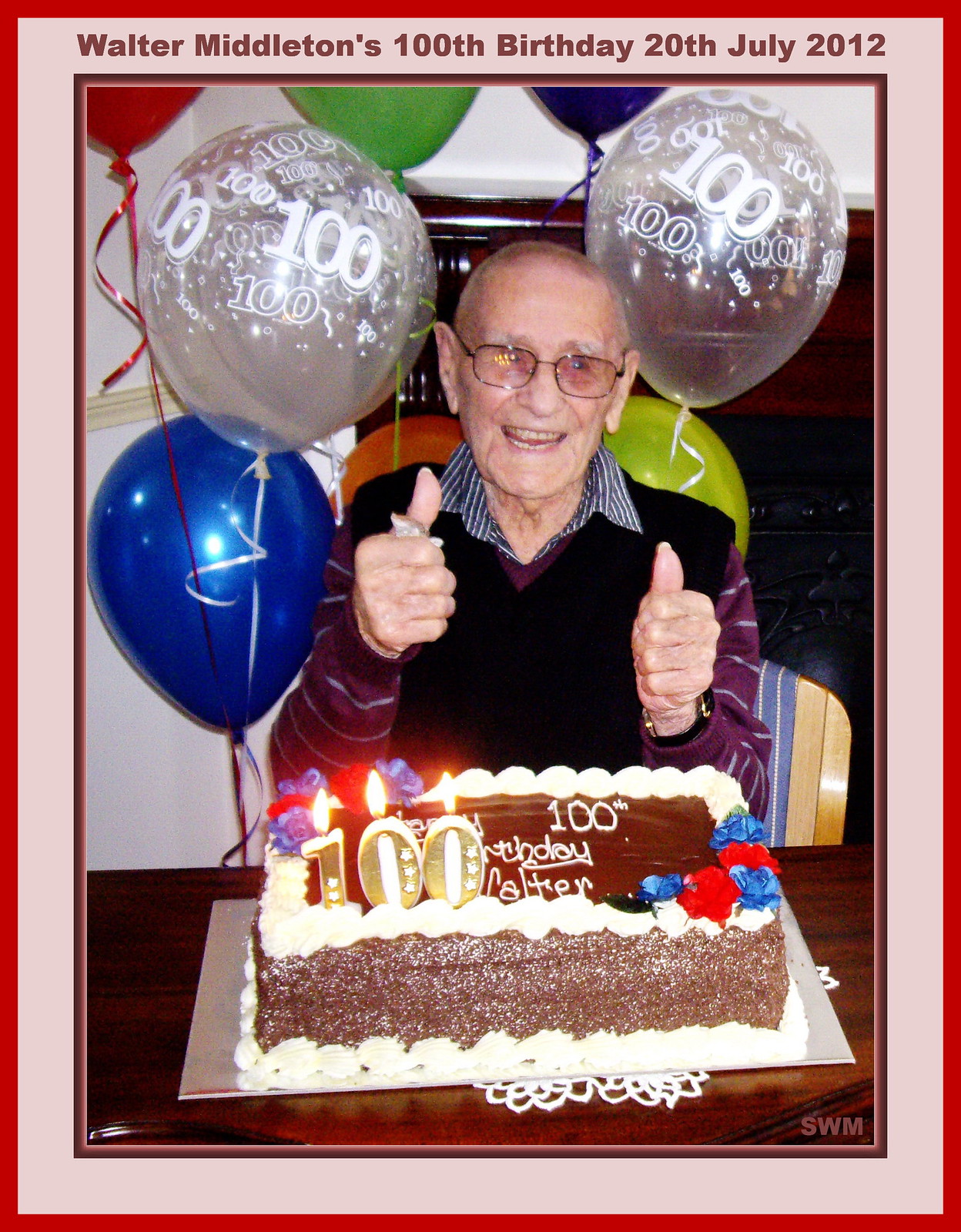Celebrating a Century: Walter Middleton beams with joy as he marks his 100th birthday on July 20, 2012. A beautifully crafted cake adorned with candles forming the number "100" takes center stage, the flames adding a warm glow to the festive atmosphere. Surrounding the cake are vibrant helium balloons in an array of colors—blue, green, orange, and red—each bearing the milestone number "100." Walter, dressed in a dark sweater vest layered over a long-sleeve purple shirt, stands beside a dark wood table embellished with red and blue floral decorations. With a jubilant thumbs up and a radiant smile, Walter epitomizes the spirit of celebration on this momentous occasion.